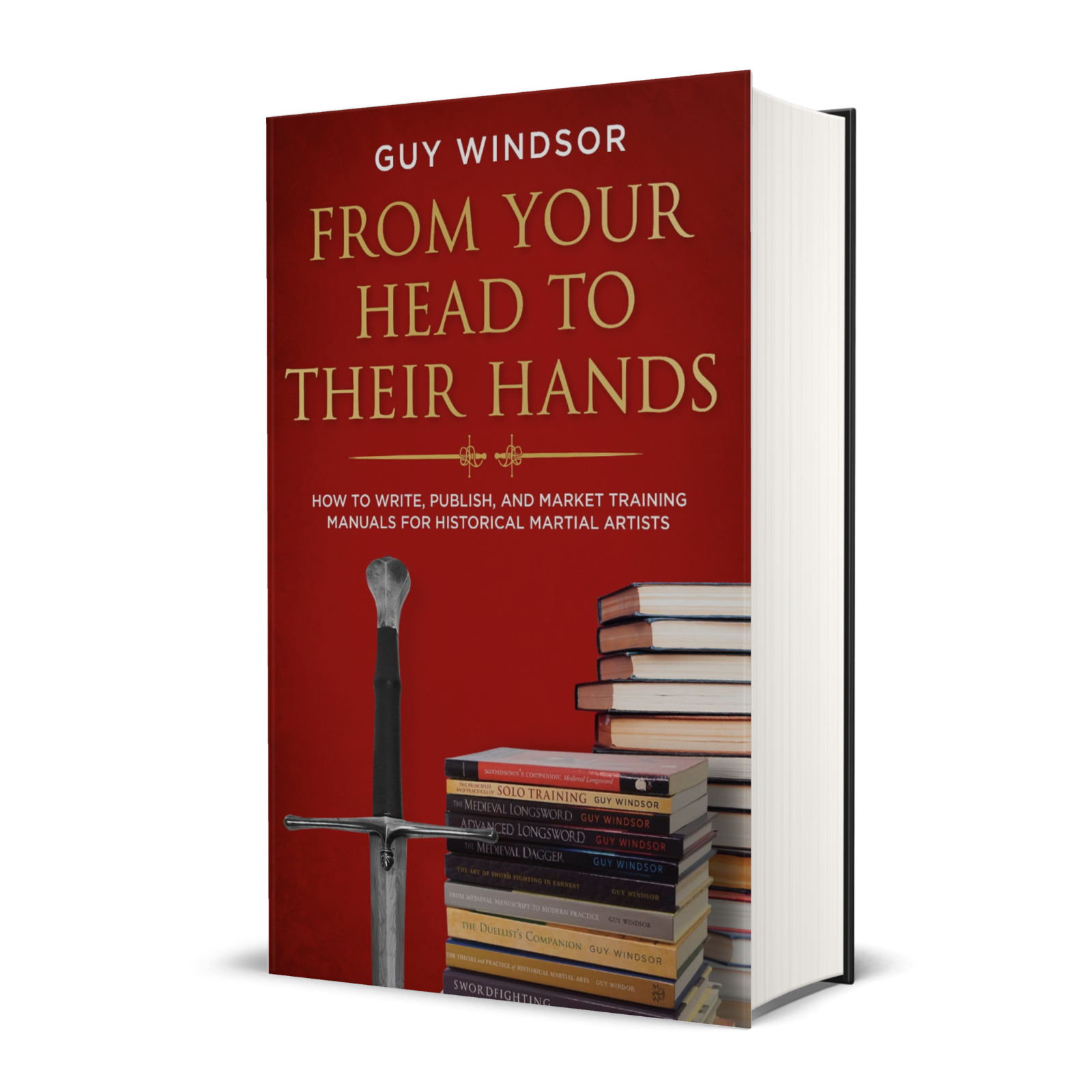The photograph captures a thick hardcover book standing upright against a stark, white background. The book has a dark reddish jacket featuring the author's name, "Guy Windsor," prominently displayed at the top in white text. Beneath the author's name, the title "From Your Head to Their Hands" is written in striking gold letters. Below this, there's more text in white that reads, "How to Write, Publish, and Market Training Manuals for Historical Martial Artists." The cover is visually rich, adorned with a detailed image showing two stacks of various books, both paperback and hardcover, along with a silver sword with a black handle positioned on the left side. Additionally, a bookmark, depicted as two swords facing opposite directions, is also visible. The pages of the book appear exceptionally white, underscoring its educational theme.